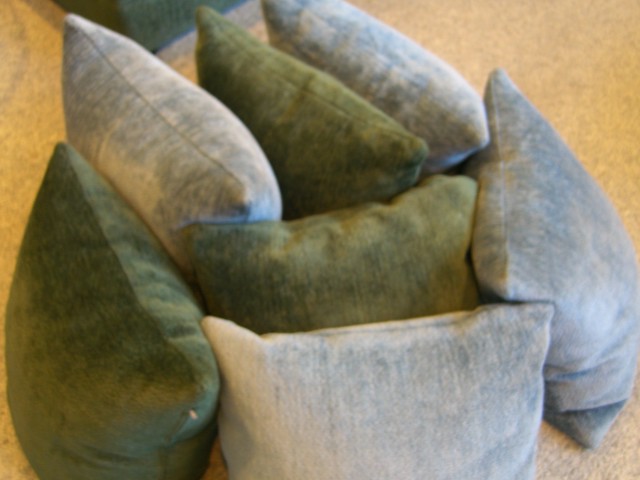The photograph depicts seven square pillows, arranged upright and closely pressed together in a near-circle formation on a cream-colored, short-fiber carpet that resembles felt. Two dark green pillows occupy the center, flanked by three blue-gray pillows – two on the right, one to their bottom, and another to the top left – with an additional green pillow to the far left. The soft lighting gives a subtle ambiance, though the image is slightly out of focus, blurring finer details. The pillows, possibly made of velveteen material, appear zipper-less, though one at the bottom left might have a zipper that is hard to distinguish. There is a glimpse of a furniture piece, likely a leg rest, intruding from the top left corner of the image. The overall scene suggests the pillows were moved, possibly during a cleaning session, and temporarily piled on the carpet.